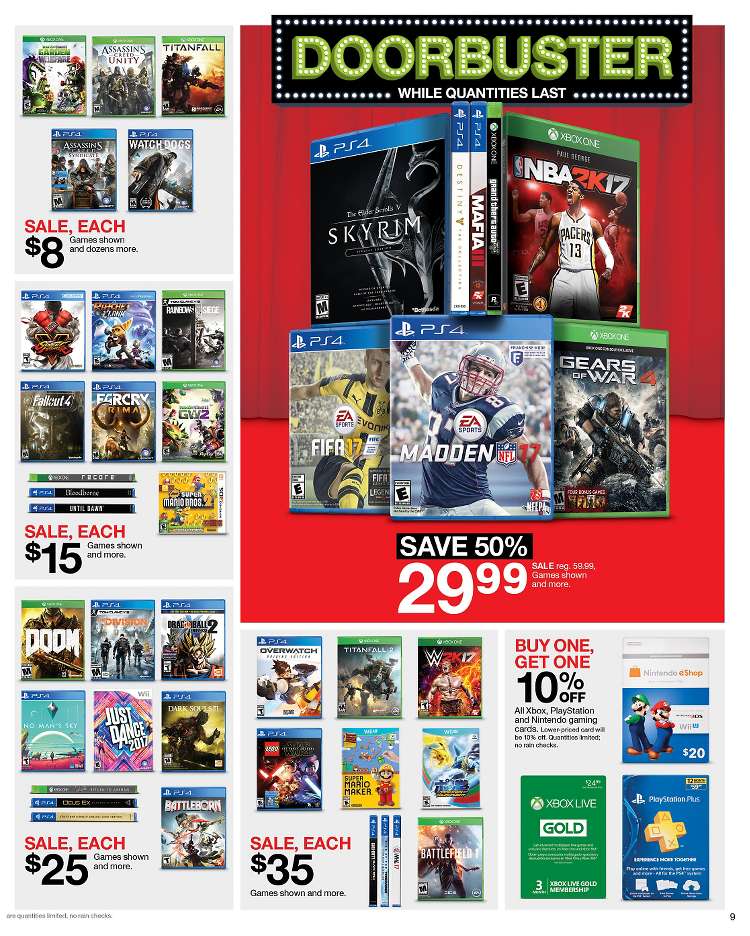This advertisement highlights doorbuster deals, likely from Target, showcasing significant discounts on a variety of video games. The layout features several sections with different price points for each set of games:

- **$8 Each:** Includes titles like *Watch Dogs*, *Assassin's Creed Syndicate*, *Assassin's Creed Unity*, *Titanfall*, and *Garden Warfare*.
- **$15 Each:** Covers games such as *Street Fighter V*, *Ratchet & Clank*, *Rainbow Six Siege*, *Far Cry Primal 4*, *ReCore*, and *Super Mario Bros. 2* on the DS.
- **$25 Each:** Features *Doom*, *The Division*, *Dragon Ball Xenoverse 2*, *Just Dance 2017*, *No Man's Sky*, *Dark Souls 2*, and *Battleport*.
- **$29.99 Each:** Lists popular titles like *Madden NFL 17*, *Gears of War 4*, *FIFA 17*, and *NBA 2K17*.
- **$35 Each:** Showcases *Overwatch*, *Titanfall 2*, *WWE 2K17*, *Pokkén Tournament*, *Super Mario Maker*, *LEGO Star Wars*, and *Battlefield 1*.

The right-hand side of the ad promotes a special offer where customers can buy one and get a second gaming card at 10% off, applicable to Xbox, PlayStation, and Nintendo gift cards, accompanied by images of these cards.